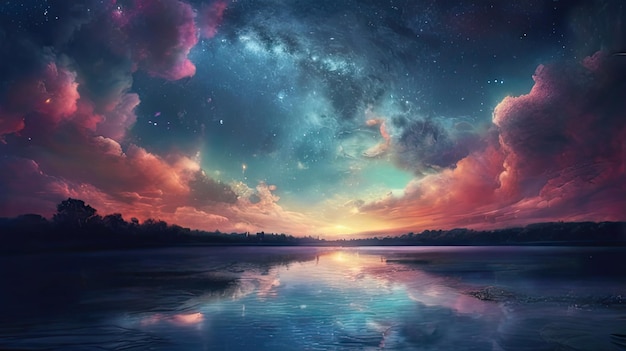The image presents a breathtaking, fantasy-esque lakeside scene rendered in beautifully striking digital art. The setting features a glistening body of water, so reflective it seems almost magical, capturing the colors of the sky in a triangular central area. The sky, transitioning from light to dark blue, is filled with fluffy clouds in shades of pink, orange, and purple, evoking the enchantment of a setting sun. Scattered twinkles of stars and suggestions of constellations or galaxies add to the celestial wonder of the night sky. 

The shoreline, shrouded in shadows and dense with trees, stretches across the horizon in silhouette, framing the scene with a sense of mystery and seclusion. Large clouds form a dramatic V pattern, drawing the eye towards the center where the vivid colors become lighter and more vibrant. The left-hand side of the horizon features towering trees, while the right-hand side shows a small mountain, both rendered in deep, dark tones against the illuminated sky. The blending of natural elements with magical hues creates an image that feels as if it could be inhabited by fairies and fantastical creatures. This skyscape beautifully captures the essence of a serene and otherworldly twilight, both on the water and above.